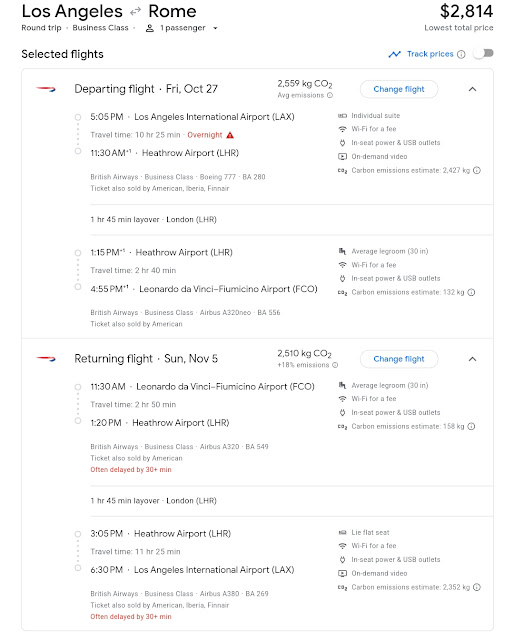A detailed screenshot of a flight booking confirmation is displayed on a computer or phone screen. The trip is a business class round trip for one passenger from Los Angeles (LAX) to Rome. The round trip is indicated by two arrows. On the right side of the screen, the total price for the trip is prominently shown as $2,814, with the note "lowest total price" in gray print below. The selected flights include the departing flight on Friday, October 27th, leaving Los Angeles International Airport at 5:05 PM. The flight duration is 10 hours and 25 minutes, and it is an overnight flight, highlighted by an exclamation point icon. The flight is operated by British Airways on a Boeing 777 aircraft. The itinerary also notes a 1 hour and 45 minute layover in London, before continuing to Rome. Further details about the return flight are listed below the departure information.